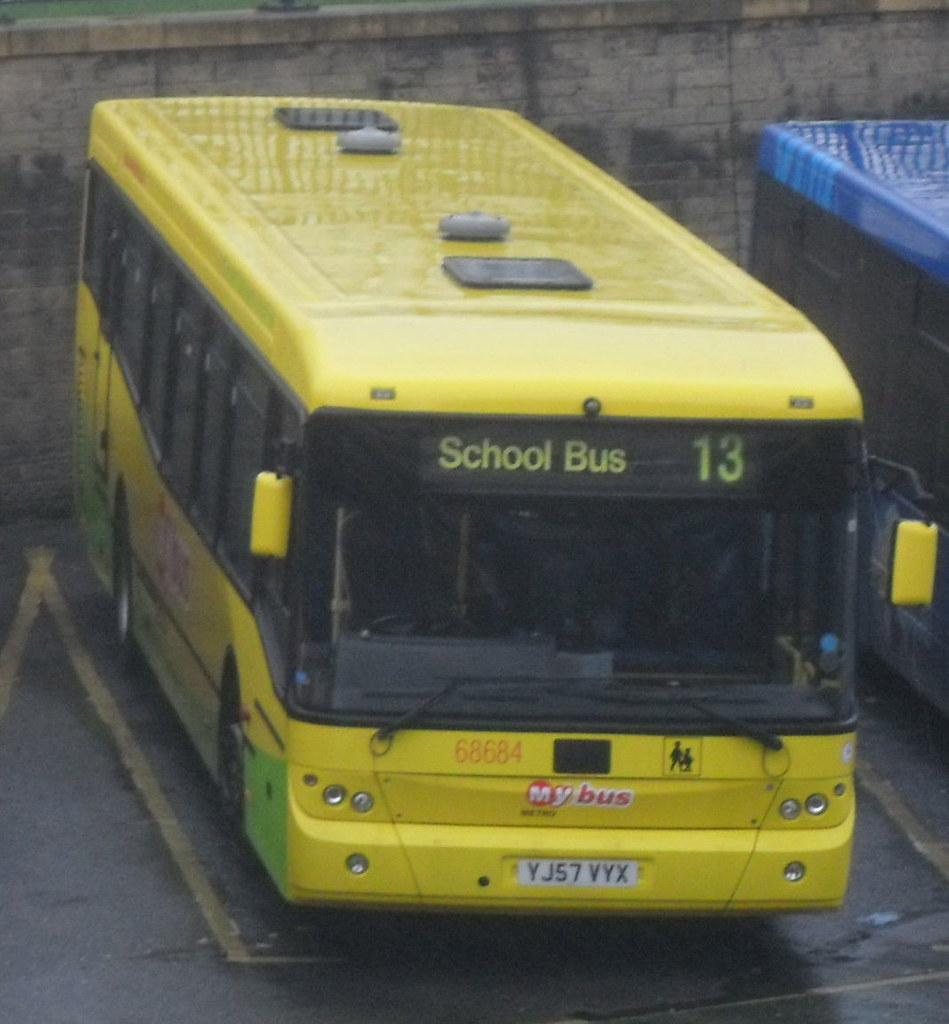This slightly grainy daylight photograph captures a vibrant yellow school bus parked in a designated spot within a parking lot. Dominating the image, the bus stands out with its shiny yellow paint, including yellow mirrors, and green accents around its bottom side. The front of the bus is adorned with the text "School Bus 13" above the windshield, while below, the number "68684" and a red "My Bus" logo are prominently displayed. The license plate, marked "YJ57VYX," sits beneath the logo. Additionally, there is a symbol on the bus portraying a person holding a child against a yellow background. The bus is parked next to another bus, noticeable by the blue-colored top at the upper right of the image. Behind the buses stretches a dirty, stained brick wall varying in shades of gray.